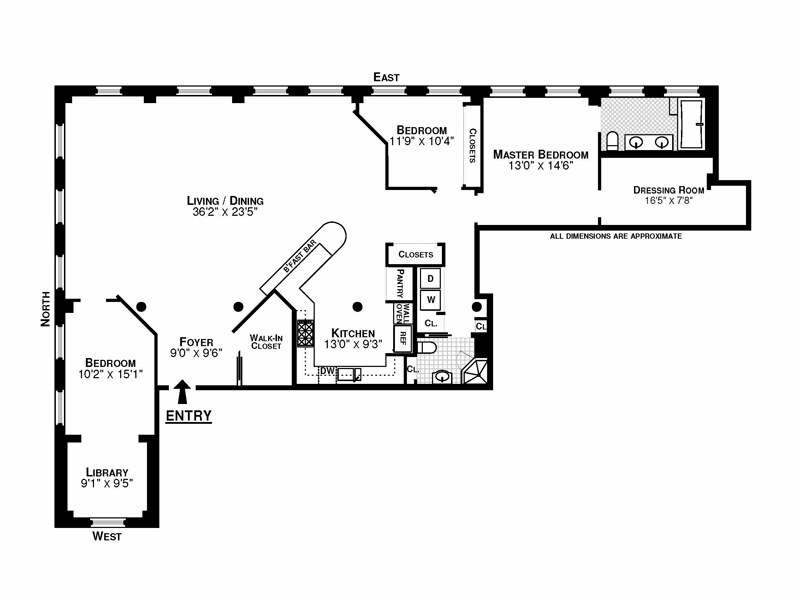This black-and-white floor plan depicts a vaguely L-shaped layout featuring various rooms that are meticulously labeled on the northern, western, and eastern extremities. The rooms include a 9' x 9' library, a 10' x 15' bedroom, and a spacious 36' x 23' living room. An equally sized 9' x 9' foyer is prominently marked, as well as a kitchen with 13' x 9' dimensions, which is positioned next to a breakfast bar and an adjoining pantry and refrigerator area. Unlabeled features include a walk-in closet and an additional closet area, as well as a bathroom. Further along, a 12' x 10' bedroom and a master bedroom measuring 13' x 14' are denoted. Adjacent to the master bedroom is a dressing room with dimensions of 16' x 8'. It is noted that all dimensions are approximate.